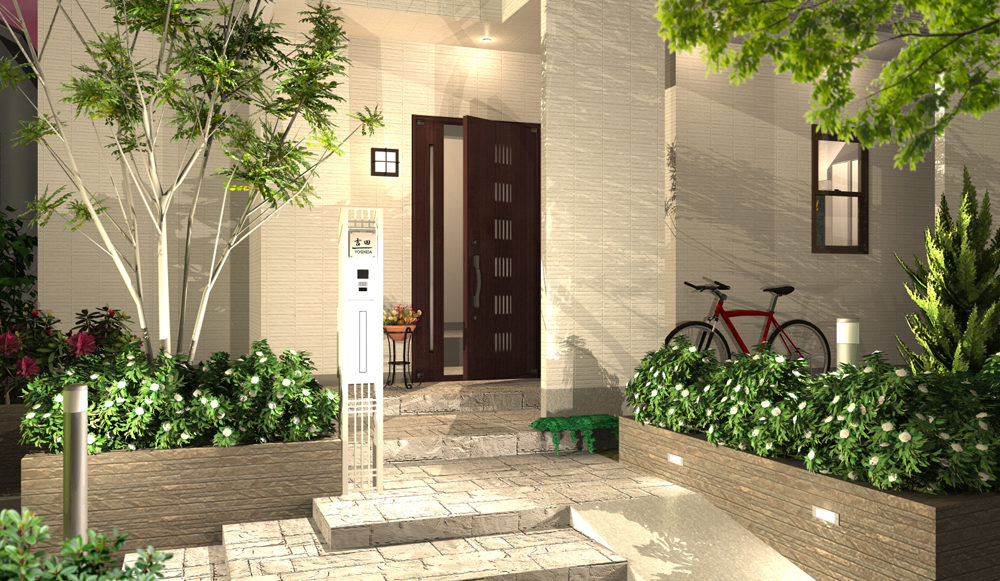The image depicts the front entrance of an upscale, white house, possibly a condo, viewed from a slightly zoomed-in perspective. The exterior features a pair of marble steps leading down from a spacious porch area. Prominent in the scene is a red, old-fashioned bicycle leaning against the right wall of the house. The front door, which is slightly ajar, is dark brown and made of wood, featuring small metal slats serving as windows. Adjacent to the door is a flower pot and a metal stand. To the front of the porch, there's a notable kiosk-like structure which might serve as a guest introduction system. Additionally, various trees, green branches, and structured shrubbery boxes add to the aesthetic appeal. The house also includes features accommodating accessibility, with steps and what appears to be a wheelchair ramp. There are also a couple of lights and a white device or pole near the entrance, possibly to prevent vehicle access. Overall, the scene combines elements that suggest both residential comfort and a touch of modern technological integration.